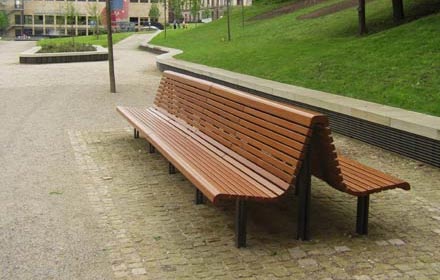In this photo, you can see a detailed park setting featuring a distinctive wooden double-sided bench. The bench is quite long, approximately 15-20 feet, and is constructed from brown wood slats that curve up to form a U-shape at the top, connecting the two back-to-back seating areas. The bench is supported by black legs, including a central pole that supports the U-shaped connection. It is placed on a neat cobblestone or brick walkway, with the walkway extending widely to the left and zigzagging off in the distance.

To the right of the bench is a small stone wall with a stone top, which borders a well-manicured grassy hill. This hill, with some tree bases visible, is part of a landscaped area that includes a raised flowerbed between two cobblestone paths and additional small gardens in the distance.

In the background, a large tan building with multiple windows can be seen, likely serving as an office or public building. This building is located in the upper left part of the image. The entire scene is framed by well-maintained green grass and landscaped areas, creating a serene and orderly park environment.